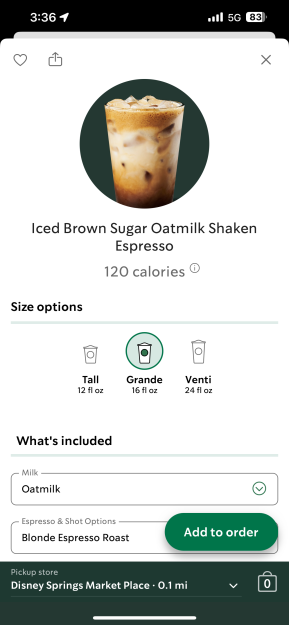This image is a mobile screenshot, possibly from a Starbucks app, featuring an ordering interface for a beverage. The top section includes the mobile status and notification bar, showing an 83% battery life, 5G network with full signal strength, and the time of 3:36, likely PM given the context. 

Central to the screenshot is a large circular image of the drink, encircled by a green border. Directly below the image, the drink is identified as an "Iced Brown Sugar Oat Milk Shaken Espresso," noted to contain 120 calories.

Further down, size options are displayed: Tall (12 fl oz), Grande (16 fl oz), and Venti (24 fl oz), with the Grande size selected for this order. The caption "What's included?" introduces the customizable options chosen: oat milk and a blonde espresso roast. 

At the bottom of the screen, a green "Add to Order" button is visible, and the pickup location is noted to be the Disney Springs Marketplace, 0.1 miles away.